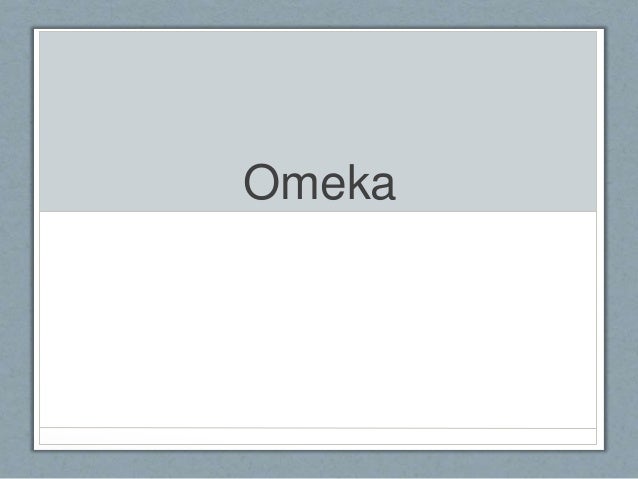The image is a slide from a slideshow presentation with a medium gray, rectangular frame. Within this frame, there is an inner rectangle divided into two halves: the top half is light gray, and the bottom half is white. The white lower half is bordered by a thin gray line. Centered in the light gray upper half of the rectangle are black letters spelling "OMEGA," with only the "O" capitalized. There is no additional text or image within the rectangle. At the very bottom of the rectangle, there are two thin gray lines running horizontally.